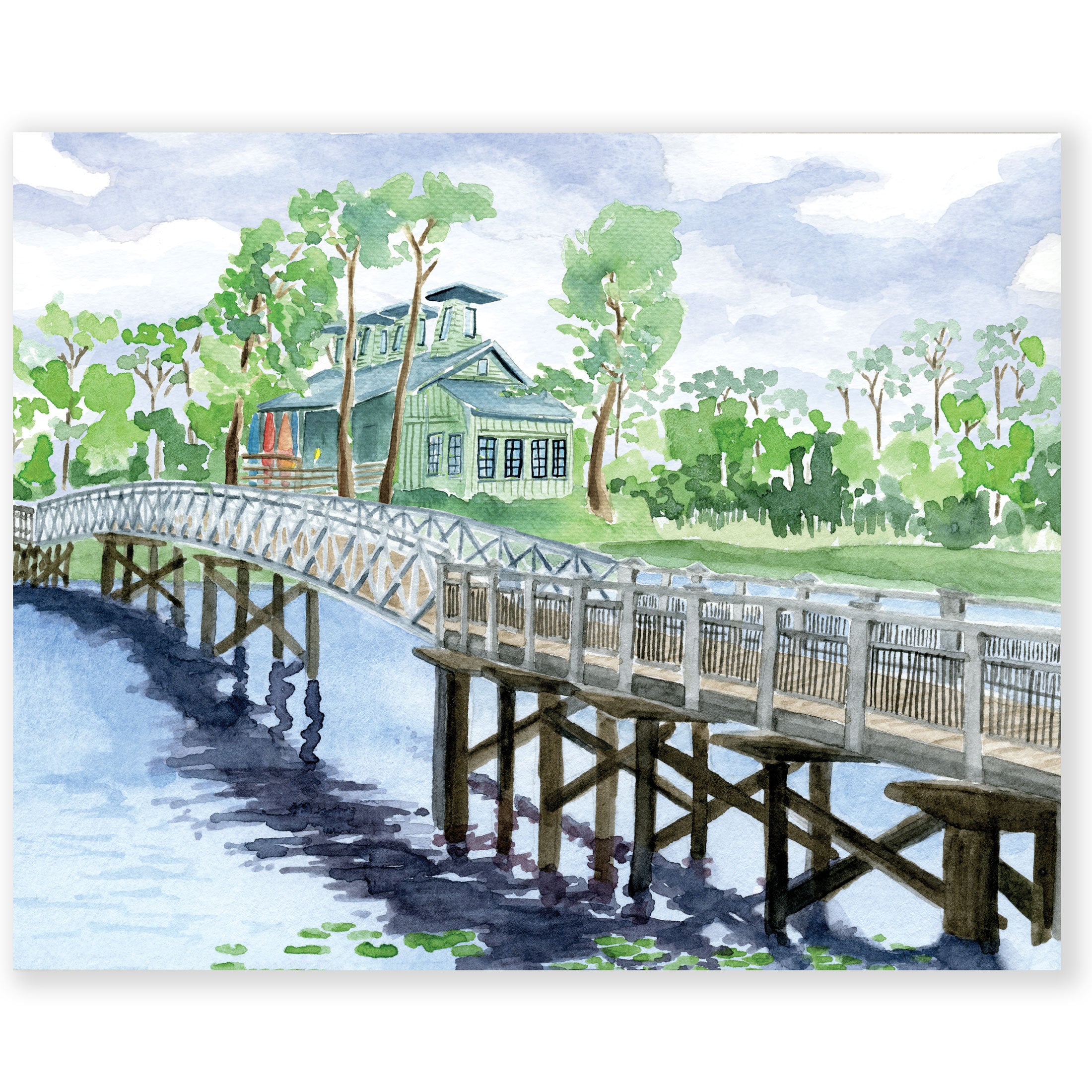This watercolor painting vividly captures a tranquil scene featuring a distinctive bridge and a house nestled among trees. The bridge, which spans horizontally across the entire painting, has sections with unique architectural details. It transitions from a straight section with silver and brown slats to an arching middle segment adorned with gray x-shaped patterns, and then back to a similar straight section. The bridge is supported by brown wooden beams that descend into the water below, casting dark blue shadows across the calm, light blue surface that is dotted with lily pads.

In the background, a green house with a gray roof, black windows, and a red door stands amidst lush greenery. The house is surrounded by an abundance of grass and vibrant trees on all sides, enhancing the serene atmosphere. Additionally, some colorful, surfboard-shaped objects can be seen near the house. The sky overhead is depicted with soft blue tones and wisps of white clouds, adding to the overall peacefulness and beauty of the scene.